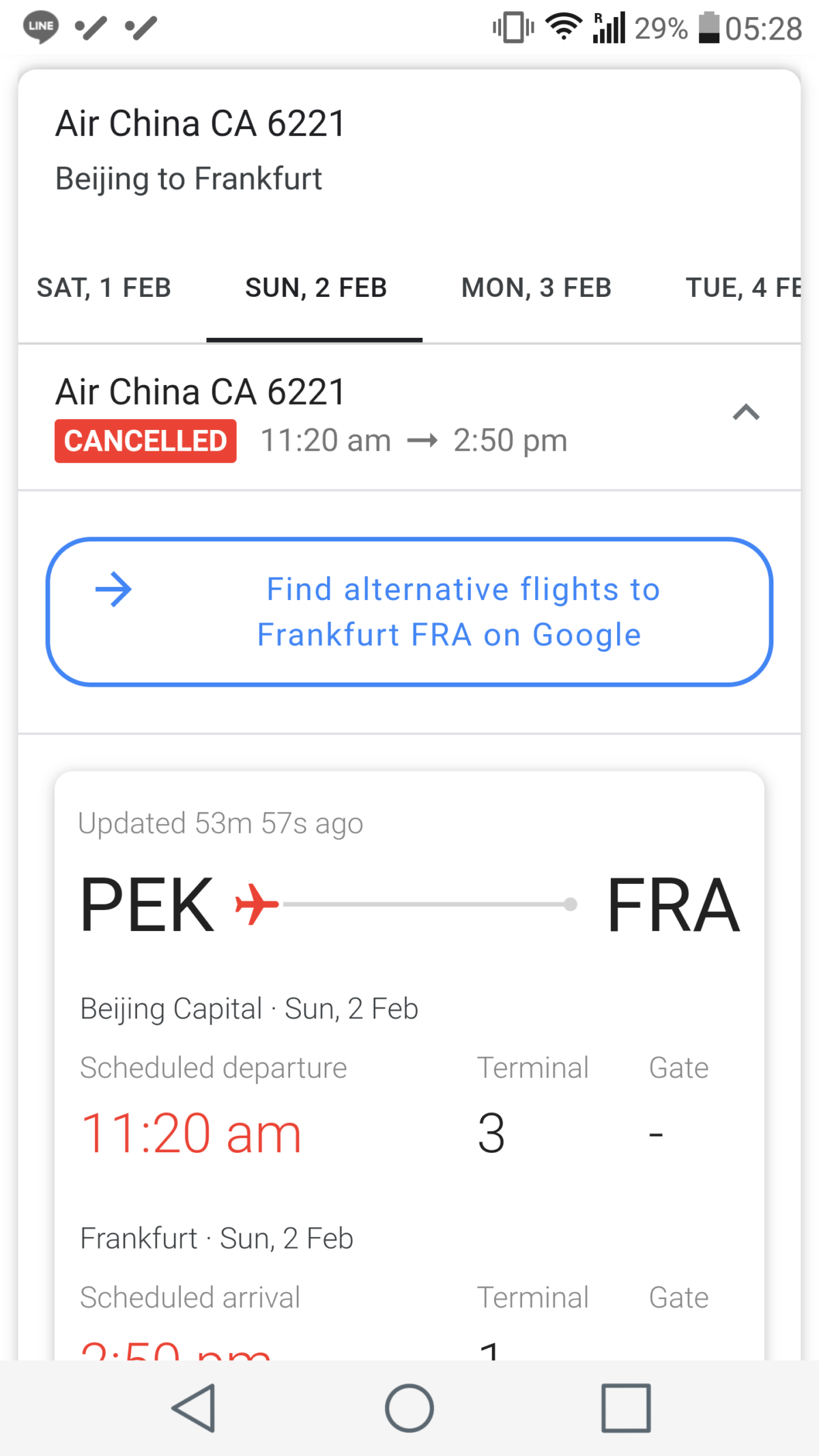Screenshot from a website displaying flight information on a white background:

- **Header:** Features a white background with a speech bubble icon in the top-left corner, containing the text "LINE" in white, capitalized letters. On the top-right, it shows a slanted diagonal dot icon followed by another similar icon, a battery at 29%, time showing 05:28, a Wi-Fi signal indicator, and a cell signal indicator.

- **Main Section:**
  - **Flight Title:** "Air China CA6221"
  - **Route:** "Beijing to Frankfurt"
  - **Navigation Bar:** Options are provided for different dates: Saturday, 1 Feb; Sunday, 2 Feb; Monday, 3 Feb; Tuesday, 4 Feb.

- **Flight Details:**
  - **Flight Number:** "Air China CA621"
  - **Status:** A red banner displays "CANCELED" in white capital letters.
  - **Times:** "1120 a.m. to 258 p.m."
  - **Alternative Flights Option:** There's a blue, outlined button with an arrow pointing right, displaying "Find alternative flights to FRA on Google" in capital letters.

- **Additional Information:**
  - **Update Timestamp:** "Updated 53 minutes and 53 seconds ago"
  - **Route Summary:** "PEK to FRA" with an accompanying red airplane icon. 
    - **Details:** 
      - **Departure:** "Beijing Capital, Sun 2 Feb, Scheduled Departure 1120 a.m., Terminal 3 Gate"
      - **Arrival:** "Frankfurt, Sunday, February 2nd, Scheduled Arrival" (content cut off)

- **Design Features:** The sections are separated with light gray borders and have a white background inside.